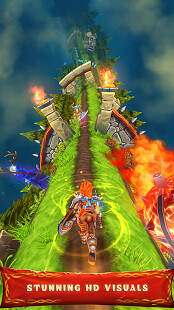The poster is vividly colored, featuring a marbled mix of blue and green at the top, creating an eye-catching backdrop. The most striking element is a prominent green streak that begins narrowly at the top and widens toward the bottom. Emanating from the left-hand side of this streak are dynamic orange flames, while the right-hand side bursts with bright blue adorned with white spots, adding to the poster's visual drama. A bold red banner stretches across the bottom, bearing the text "Stunning HD Visuals" in a way that commands attention. In the background, a circular brown object is subtly illuminated with lights, though it's challenging to discern whether it represents a creature or another form. The overall composition is visually arresting and richly detailed, drawing the viewer into its vibrant, intricate world.